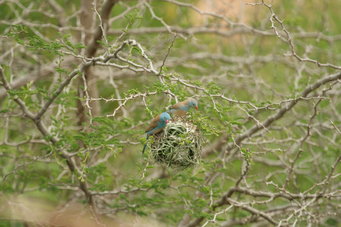The photo features a close-up of thin, frail, and grayish-brown dead tree branches, devoid of leaves. In the midst of these branches, nestled at a lower height akin to a shrub or hedge, is a bird's nest. This nest is circular, composed of green, brown, and a touch of white materials. It houses two birds, which could be interpreted as a couple or merely companions. These birds are vividly colored with blue heads and chests, brown wings, and one possibly having an orange beak. The scene hints at the arrival of spring; sparse green leaves are just beginning to appear in the background, suggesting new growth. The ground beneath consists of green grass, potentially indicating a transitional phase with some patches appearing more verdant than others. The lighting suggests mid-day, capturing a serene moment in natural light. A slight blur in the bottom left corner hints at a possible obstruction like a finger close to the camera lens.